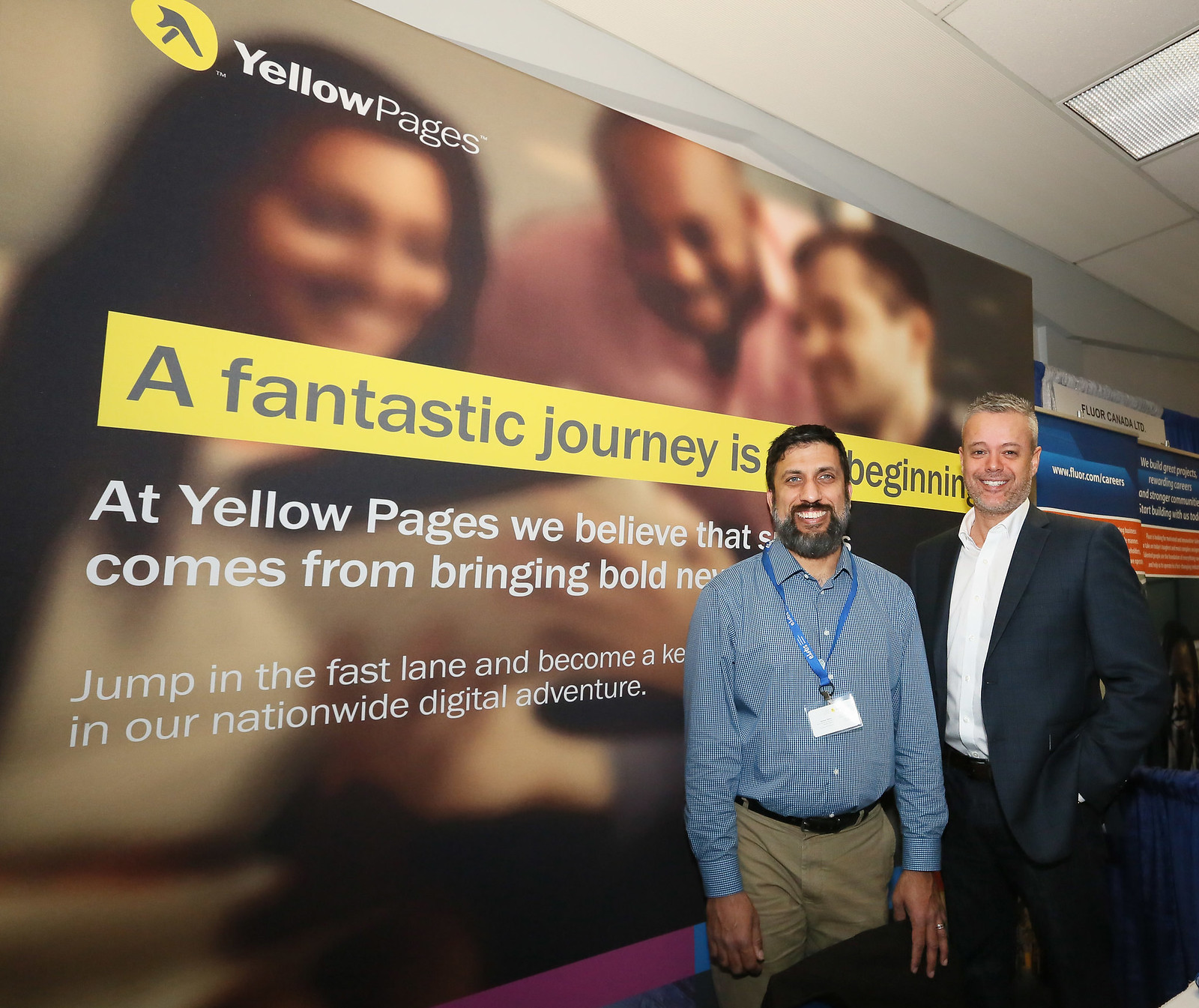Two formally dressed men are standing side by side and smiling warmly at the camera in front of a large, partially obscured sign. The man on the right is wearing a dark blue blazer over a white shirt, has short, gelled, gray hair, and has his hands in his pockets. To his left, the man is clad in a blue and white plaid shirt, accompanied by a blue lanyard with a white badge, tan pants secured with a black belt, and he sports a black and gray beard. His hands are positioned at his sides, one resting on a chair. The sign behind them, featuring a yellow banner with the slogan "A fantastic journey is beginning" prominently displayed, partially obscured by the second man, promotes Yellow Pages. The slogan continues with motivational phrases like "We believe that bold moves bring remarkable change," and "Jump in the fast lane and become a key part of our nationwide digital adventure." The background is slightly blurry but depicts a woman in white clothing, possibly holding a baby, along with other figures, while the top left corner of the image exhibits a Yellow Pages logo—a yellow oval encasing an 'A' shape made from two black lines.